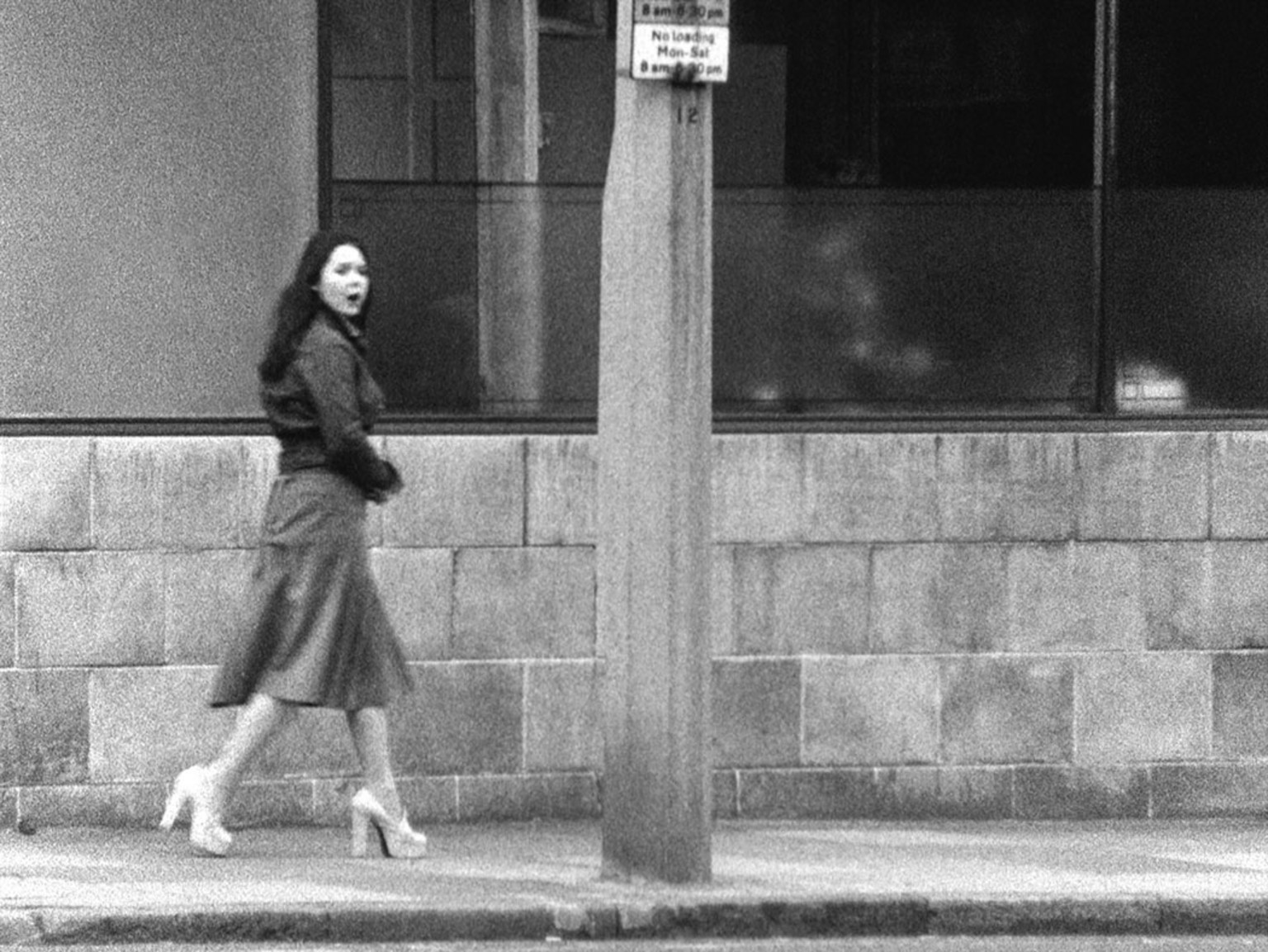This square, black-and-white photograph captures a young woman walking outdoors in the daytime, illuminated by natural light. With long dark hair cascading halfway down her back, she is depicted in profile as she strides towards the right, glancing over her shoulder at the camera. She wears a dark-colored top, a gray skirt, and striking white platform heels with thick soles. The setting includes a concrete lamppost and a building with a waist-high wall of cinder blocks patterned like bricks. Above the wall are frosted windows, indicative of a possible diner or restaurant. A small curb runs along the bottom of the image, adding to the street scene ambience. The seemingly candid moment is rich with texture and detail, balanced by the juxtaposition of the woman's poised figure against the stark architecture.